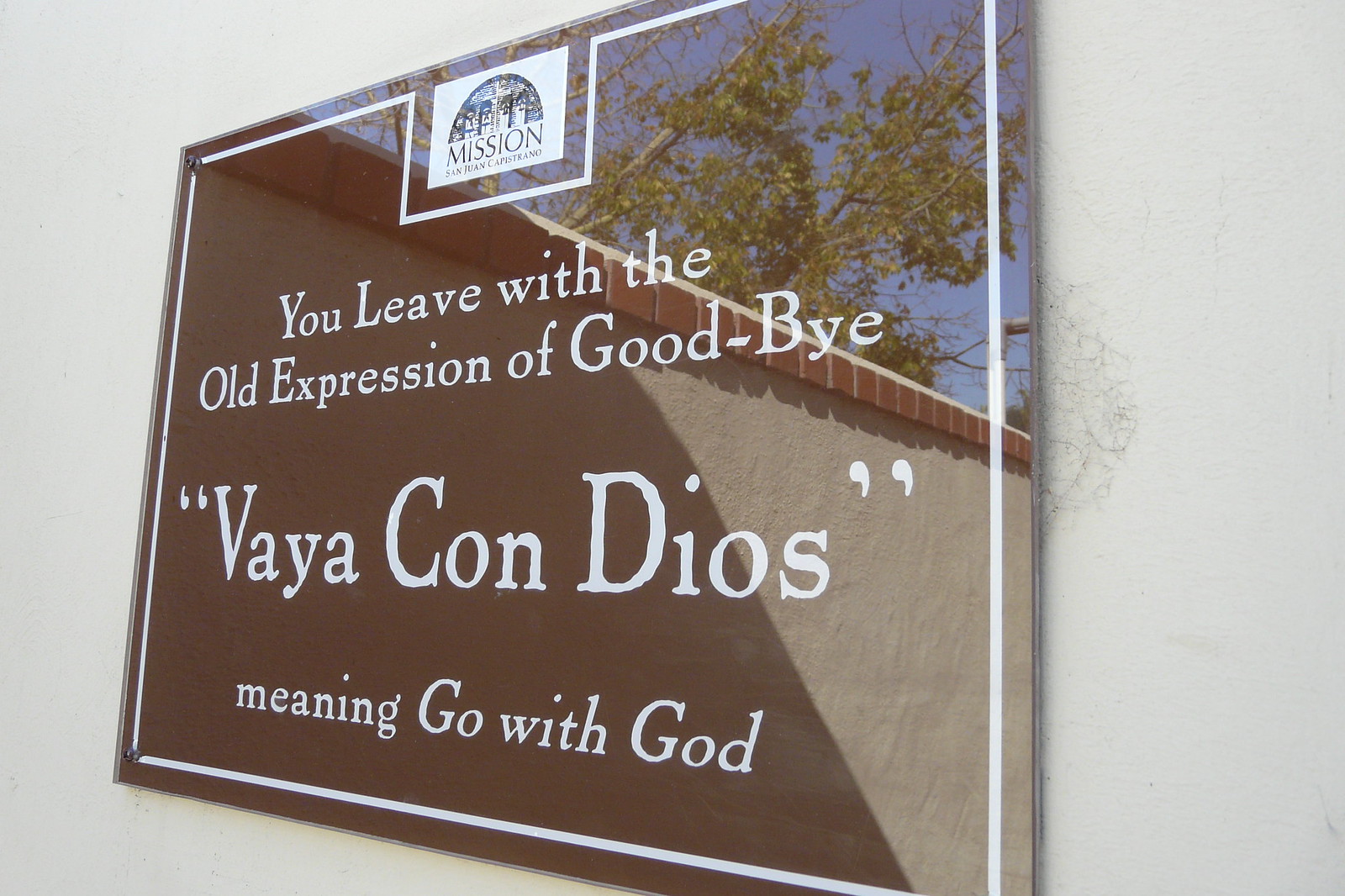The image captures a reflective, glossy black plaque affixed to an aged, off-white textured wall. The photograph is taken from an angle, highlighting the mirrored surface of the plaque, which reflects nearby elements like the wall opposite, trees with sprawling branches, and a section of the skyline. The top of the plaque features a prominent mission logo, set within a white border that frames the entire sign. Below the logo, in white text, the plaque reads, "You leave with the old expression of goodbye." In larger, bold letters, the phrase "Vaya con Dios," meaning "Go with God," is quoted. The wall's reflective nature and the detailed inscriptions create a striking contrast against its weathered backdrop.